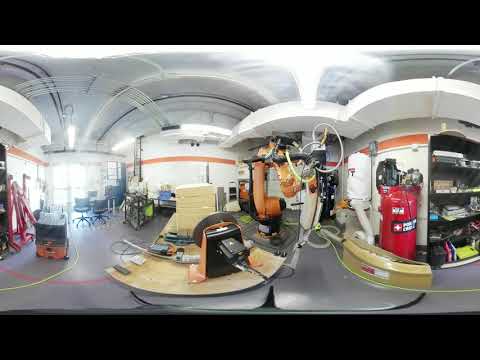The image depicts the interior of a bright, white robotics lab, captured with a fisheye lens for a wide perspective. The central feature of the lab is a substantial orange tube, almost the size of a human torso, which appears to be part of a large robotic arm. To its left, there is a stack of foam. On the right, a tall red gas tank approximately four feet high stands prominently beside a white tank on the wall, from which white tubes extend. Further to the right, a black bookcase is filled with various items. Office chairs with black rolling bases are situated near windows on the left side, allowing plenty of natural light to flood the lab, supplementing the ceiling's interior lighting. A machine with a cord sits on a desk in the foreground, and an expansive door to the left lets in additional light, contributing to the overall brightness of the space.